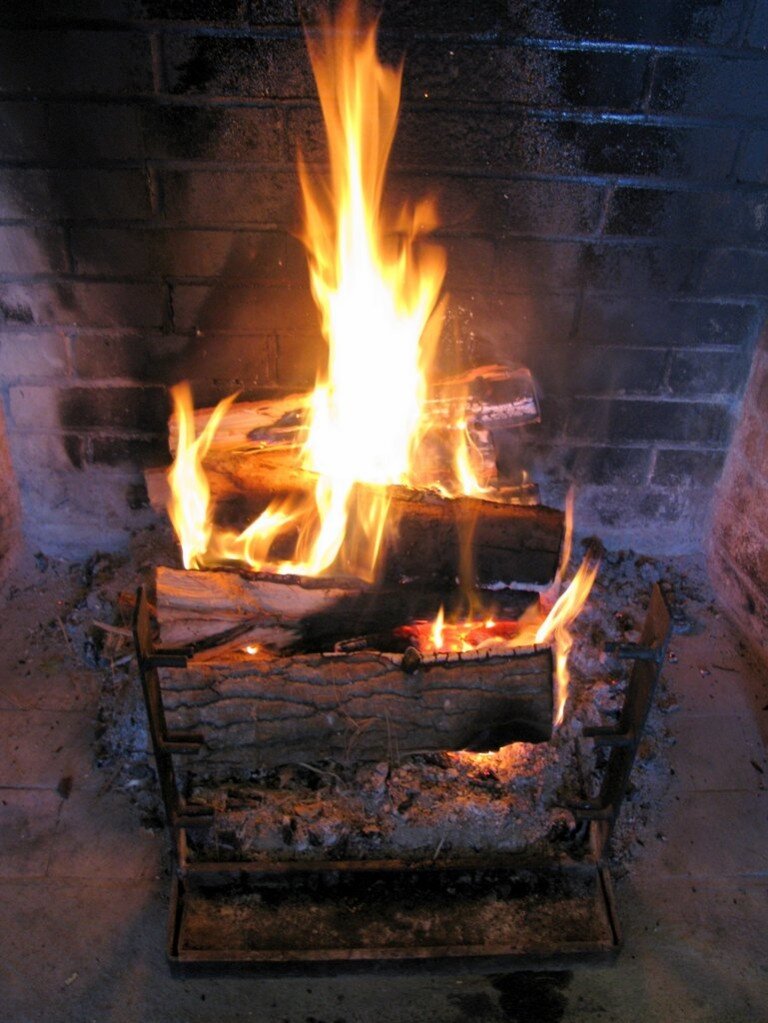This indoor photograph captures a fireplace area, viewed from above, with dimensions approximately five to six inches in height and four inches in width. The upper half of the image features the back of the fireplace, constructed from horizontal bricks now blackened from soot, transitioning into gray ash lower down. The side walls of the fireplace are still visibly brown, contrasting with the ashy bottom. Central to the image is a black fire grate holding five stacked logs in varying shades of gray and black. These logs are actively burning, emitting a bright, almost white flame at the center, with orange tips. The surrounding area is sprinkled with white ash and debris, contributing to a slightly noisy and blurry image quality, indicative of a dimly lit indoor setting.